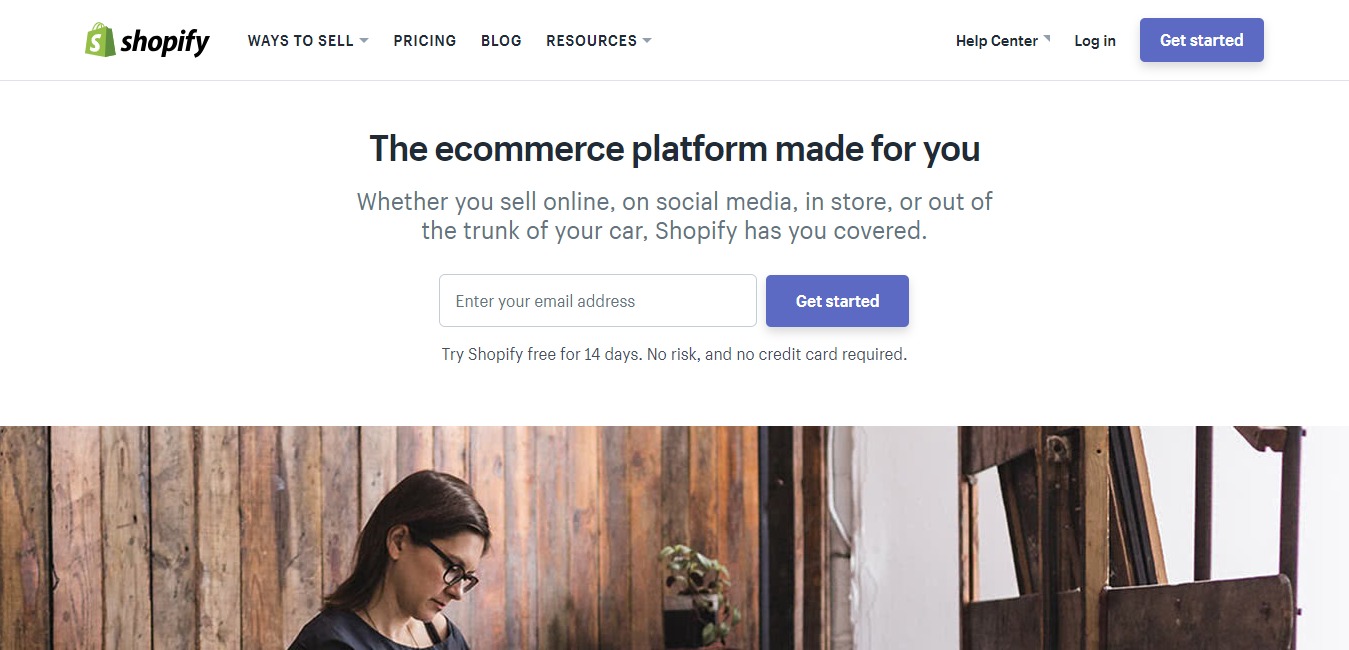This image is a screenshot from the Shopify website. In the top left corner, the black Shopify logo is clearly visible next to a green shopping bag icon with a white "S" in the center. Adjacent to the logo, several navigation options are lined up horizontally: "Ways to Sell," "Pricing," "Blog," and "Resources." On the top right-hand corner, more options are listed, including "Help Center," "Log In," and "Get Started."

Dominating the center of the webpage is a bold, black title that reads, "The eCommerce Platform Made for You." Beneath this title, a description outlines the platform's versatility, stating, "Whether you sell online, on social media, in a store, or out of the trunk of your car, Shopify has you covered." Directly below this statement, there is a field where users can enter their email address to get started with Shopify.

At the bottom of the page, there is an image of a woman with dark brown hair and black glasses, looking downward, adding a personal touch to the website's professional appearance.